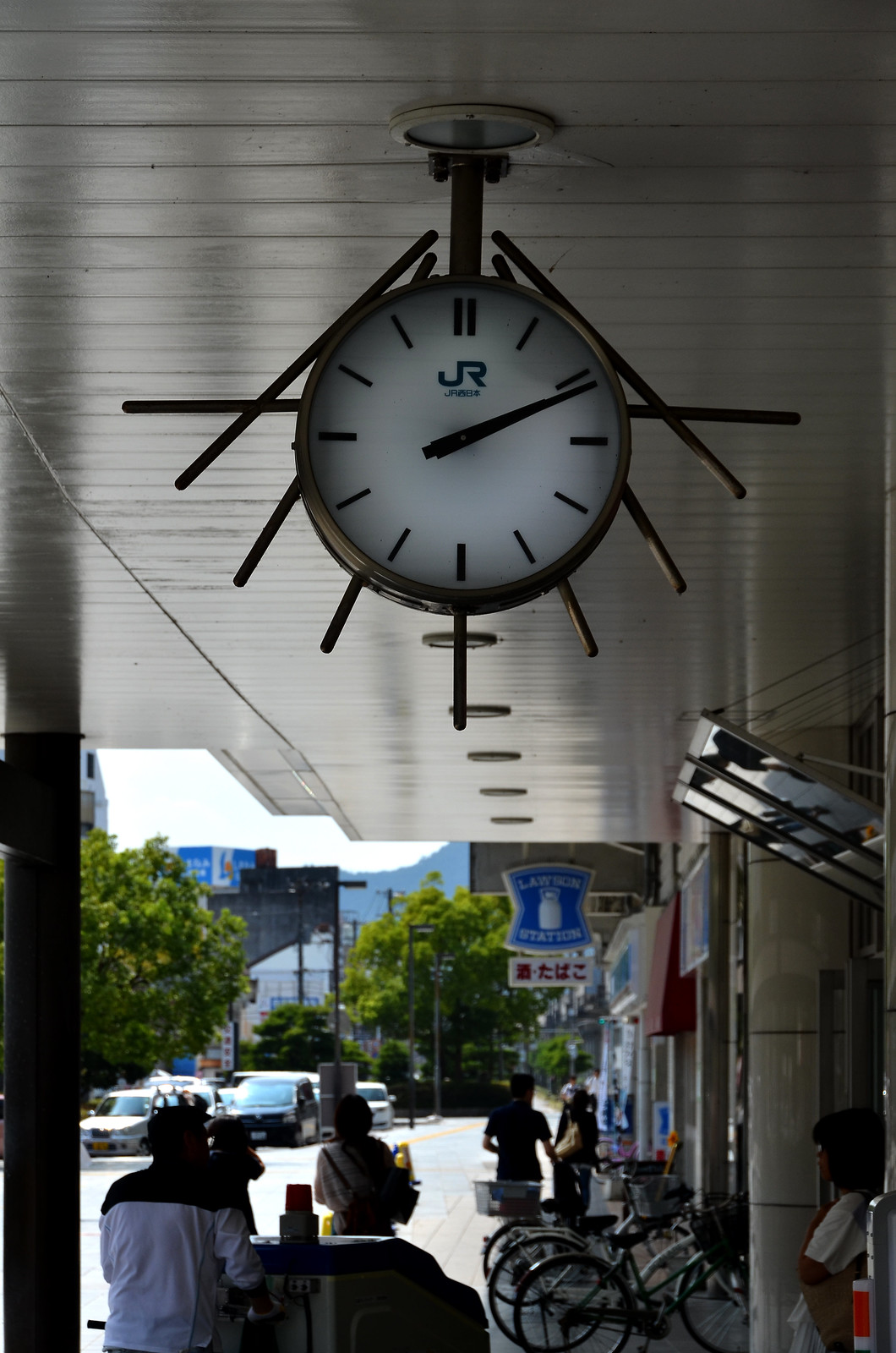The image captures a bustling outdoor scene brimming with activity. On the right side, a row of stores is visible, each adorned with various signs, one of which reads "something station." A prominent white sign with oriental letters adds to the area's multicultural vibe. A large open window is noticeable on the right, with an individual standing in front of it, possibly a customer or store employee. Several bicycles are parked nearby, highlighting the pedestrian-friendly nature of the area.

Above the stores, a white awning stretches out, providing shelter for passersby. Attached to the awning is a striking clock mounted on a silver pole. The clock features a white face with minimalist lines representing the numbers 1 through 12, with a double line denoting the 12. The logo "JR" is visible beneath the numbers, though the smaller text below it is unreadable. The clock's black minute and hour hands indicate the time is 12 past 2. Surrounding the clock are several black bars extending outward like spokes, adding a decorative element to the timepiece.

In the background, the urban landscape extends to several multi-story buildings, including a notable blue structure in the distance. A large tree is positioned to the left, partly concealing yet complementing the buildings behind it. The street in the foreground is marked with a yellow line, with cars proceeding towards the viewer, emphasizing the city's dynamic flow.

A potential food stand is situated in the bottom left corner, somewhat shadowed. Here, a man with his back facing the camera is discernible, dressed in a white long-sleeved shirt accented with black from the neck to the shoulders. He appears to be pushing a cart, possibly laden with cups or similar items. Pedestrians move across the scene, some passing by the man and others in front of the stores, adding to the lively atmosphere of the snapshot.